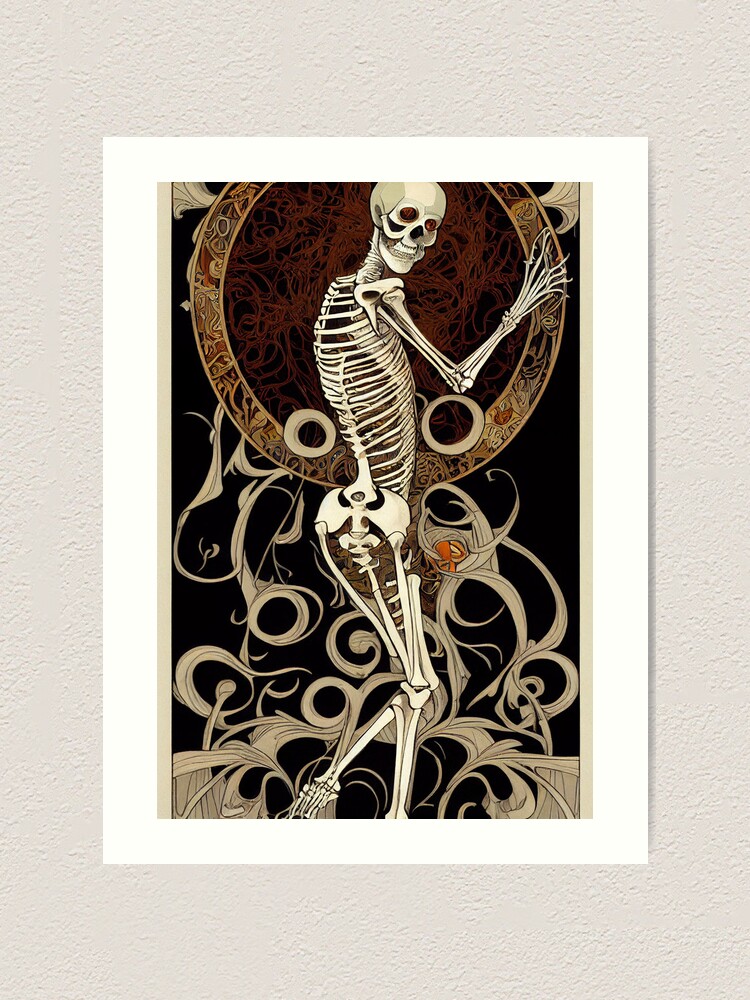The image is a detailed artwork of a human skeleton standing against a dark black background, possibly resembling the back of a tarot card. The skeleton is posed casually in profile, with its face turned and smiling at the viewer, displaying prominent teeth and striking red eyes. It has its right arm bent at the elbow, reaching upwards towards a circular metallic object. The hand, intriguingly, resembles tree branches rather than bones. The skeleton stands on one leg with the back leg bent at a 45-degree angle, adding to its relaxed demeanor. Notably, the rib cage is remarkably exaggerated, with an abundance of ribs extending almost down to its knees. Surrounding the skeleton is a circle featuring intricate designs, with a tan outline and red, squiggly lines filling the center. The lower part of the image is accented with gray, swirling lines that rise from the bottom left and right sides, merging into the composition and adding a touch of dynamic movement to the scene.